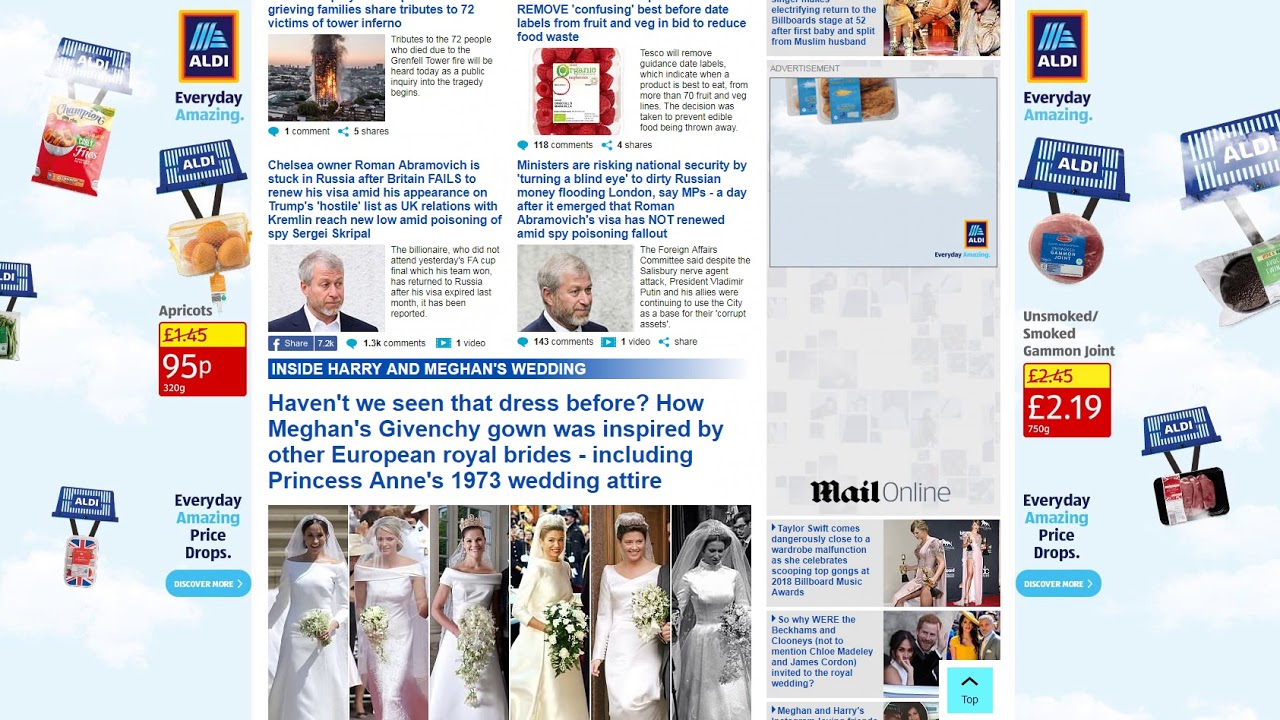The screenshot from the web page showcases a mixed layout of news articles and advertisements. Dominating the visual space are multiple Aldi ads, prominently featuring vibrant products such as snacks, apricots for 95 pence, and unsmoked/smoked gammon joint priced at 2 pounds and 19 pence, all under the slogan "Everyday Amazing." These advertisements employ striking colors, notably blue and red, to draw attention.

In the center of the page are various news articles presented in a more subdued, neutral tone, with bold headlines and a layout designed for easy scanning. The articles include a poignant tribute to the 72 victims of the Grenfell Tower fire, accompanied by a stark image of the burning building. Another piece covers Roman Abramovich's visa complications, with his image illustrating the discussion. Further topics include concerns over national security risks linked to "dirty Russian money" in London by MPs, including Abramovich's visa status.

There is also a special feature on Meghan Markle's wedding gown, comparing it to other royal brides, enriched with multiple images. The overall layout strategically places ads on the sides and keeps the news articles in the center, ensuring readability through black text on a white background.

In summary, the web page effectively combines commercial advertisements with news content, utilizing bold headlines and vibrant visuals to capture the reader's attention.